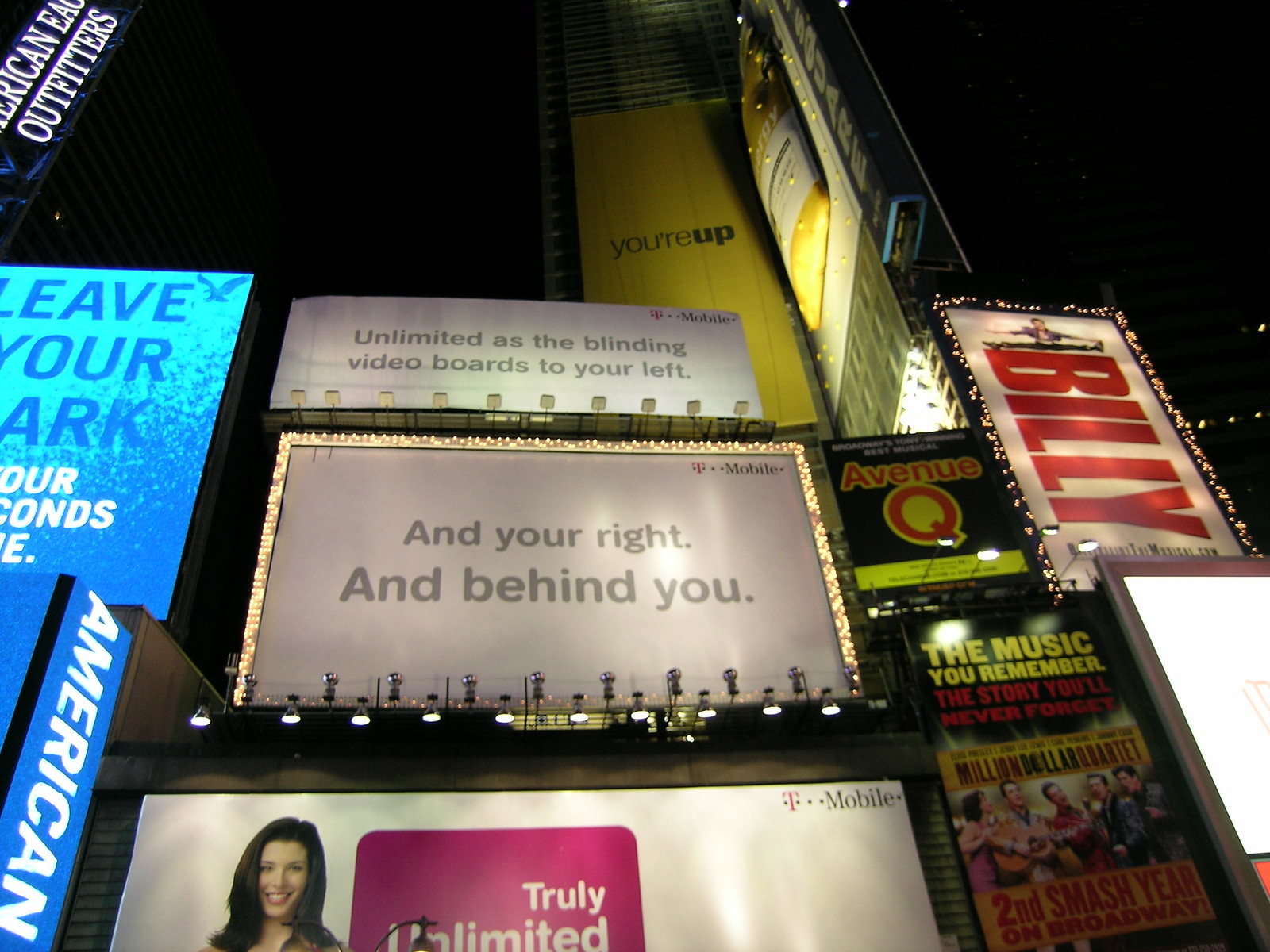This photograph, taken from the ground in an urban theater district likely resembling downtown New York City, showcases a vibrant array of illuminated billboards set against a dark night sky. Prominently featuring multiple signs, the photo's central focus is a gold-framed T-Mobile billboard proclaiming, "And you're right, and behind you." Just above it, a white rectangular sign reads, "Unlimited as the blinding video boards to your left," emphasizing the pervasive glow of the surrounding advertisements. At the very bottom, another T-Mobile billboard displays, "Truly Unlimited," featuring a dark-haired, light-skinned woman with a big smile beside a purple square. Adjacent to these central advertisements, to the right, is a neon sign for American Eagle Outfitters, while another sign for the Broadway musical Billy depicts a performer in a mid-air split. The entire scene is punctuated by the brightness of these signs, reflecting off the night sky and creating an iconic urban tapestry.